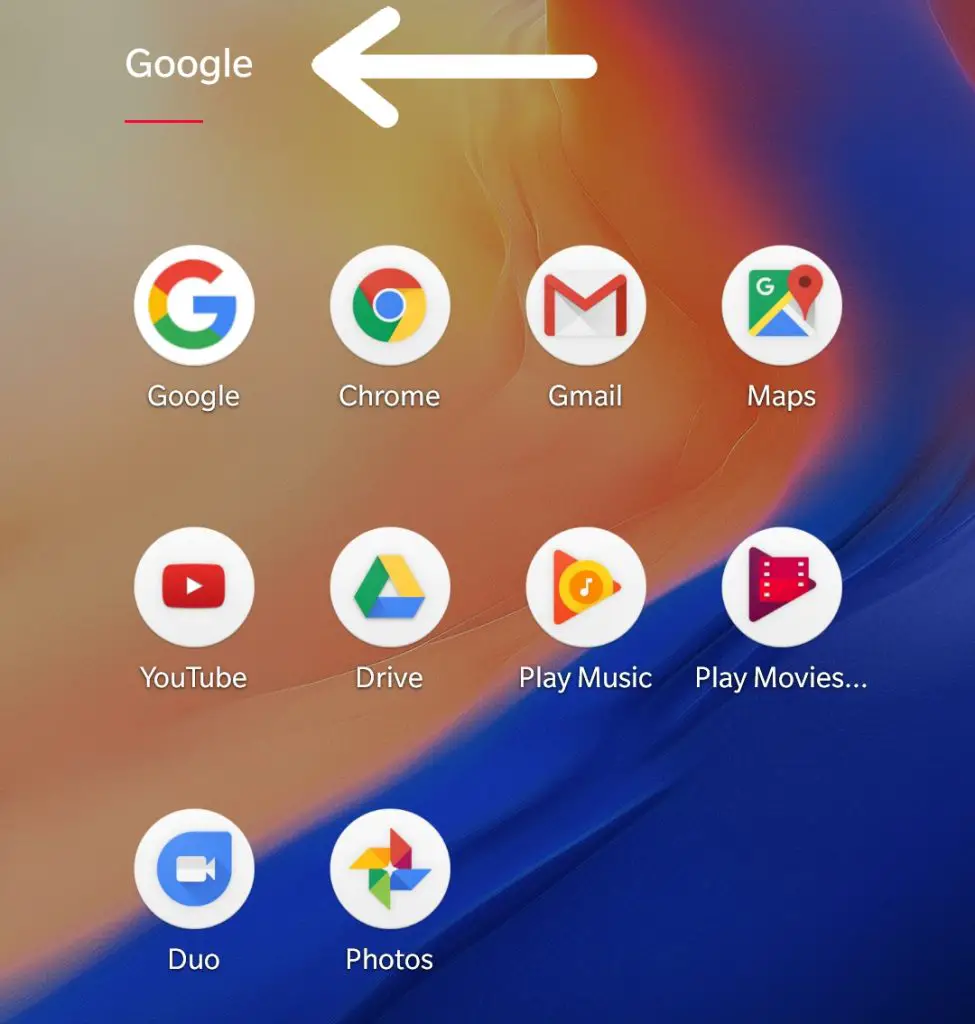The image prominently features various Google apps displayed on a white background, with a large white arrow pointing towards the word "Google." Each app icon is distinctly recognizable. 

1. **Google**: Displayed with the characteristic "Google" lettering in red, yellow, green, and blue.
2. **Google Chrome**: The icon features the Chrome logo with a blue circle center, surrounded by segments of red, yellow, and green. The word "Chrome" is written at the bottom.
3. **Gmail**: Recognizable by its white envelope icon outlined in red.
4. **Google Maps**: Features a multi-colored pin with sections of green, blue, red, and yellow.
5. **YouTube**: Shows a red rectangle with a white play triangle in the center. The name "YouTube" is at the bottom.
6. **Google Drive**: Depicted with a triangular logo composed of green, yellow, and blue segments, and labeled "Drive" below.
7. **Google Play Music**: The icon is an orange triangle with concentric circles in orange hues, featuring a white musical note inside. The text reads "Play Music."
8. **Google Play Movies**: This icon has a dark burgundy triangle resembling a movie reel with a gradient effect, labeled "Play Movies."
9. **Google Duo**: A blue, diagonal teardrop shape with a white camera inside.
10. **Google Photos**: Shows a pinwheel or flower-like arrangement in yellow, green, blue, and red, labeled "Photos."

Together, these icons depict a comprehensive suite of Google's applications with their distinctive designs and colors, all set against a clean white background.